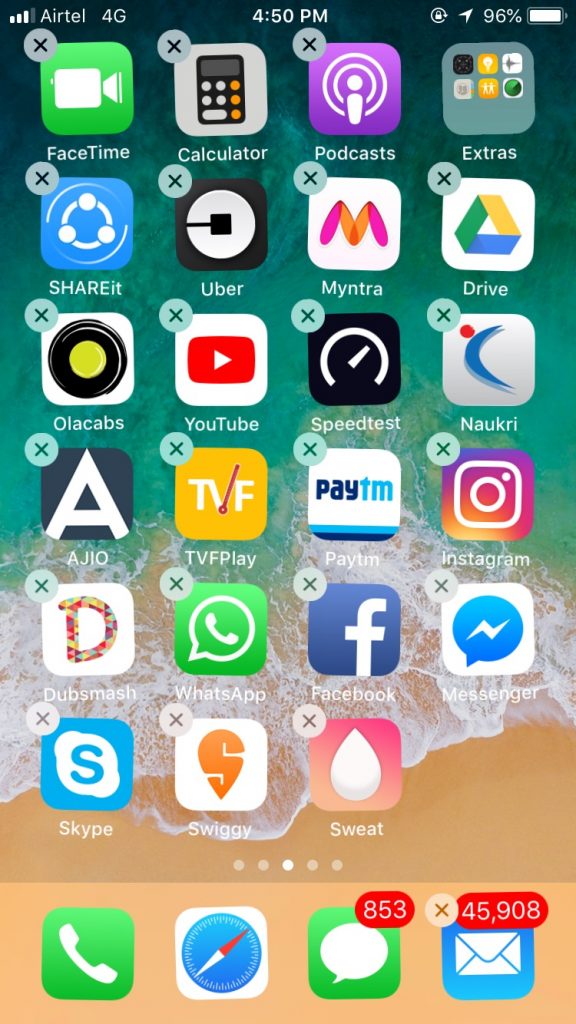A detailed and cleaned-up caption for the image could be:

"A screenshot of an iPhone home screen taken at 4:50 p.m. At the top center, the time is displayed. The first row of app icons includes FaceTime, Calculator, Podcasts, and a folder labeled 'Extras' which contains Find My Phone, Contacts, and Voice Memos. The second row features ShareIt, Uber, Mantra, and Google Drive. Moving to the third row, there are VLC player apps, YouTube, Speedtest, and an app called Naukri. Following that, the fourth row includes Chill TV, FPlay, an ATM app, and Instagram. The fifth row comprises Dubsmash, WhatsApp, Facebook Messenger, Skype, Swiggy, and an app named Sweat. Lastly, the dock at the bottom shows the Phone, Safari, Messages, and Mail apps."